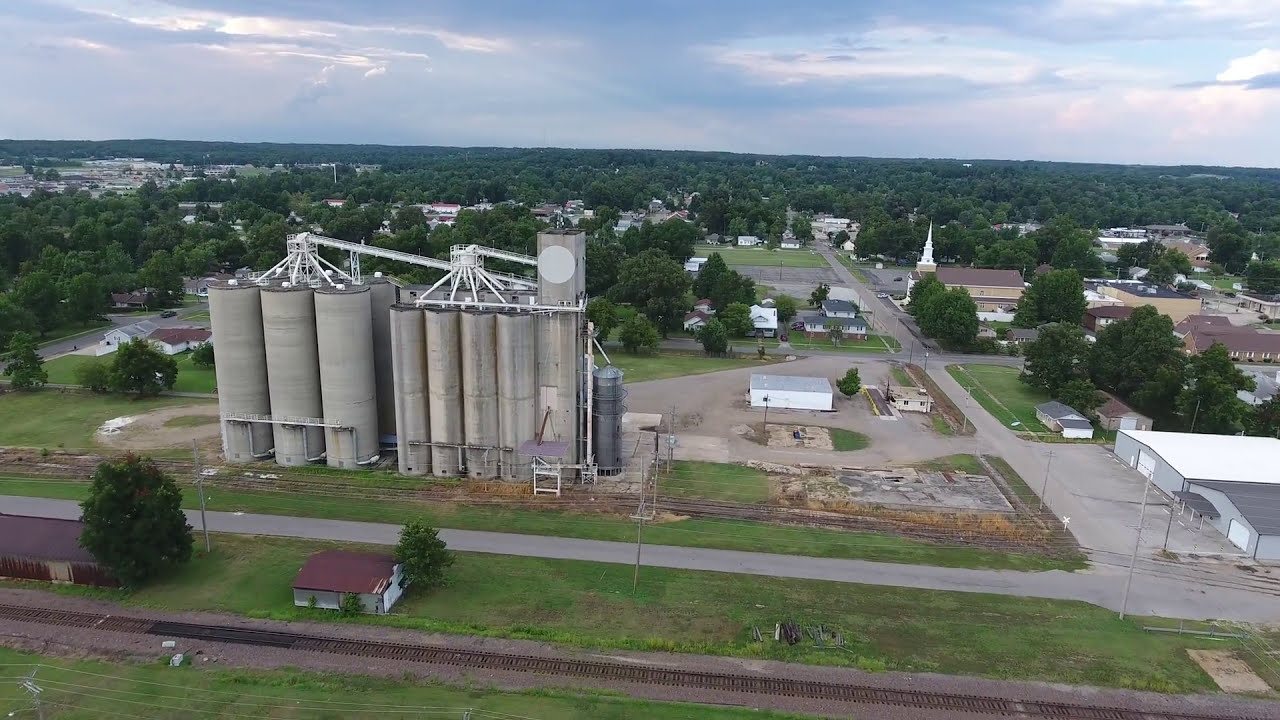This detailed aerial photograph captures a small town or farm town taken from an elevated viewpoint. The central focus is a green industrial building or mill, prominently featuring multiple cylindrical cement silos on the center left. Surrounding this structure, the ground is mostly covered with green grass, with additional green trees both behind and dotted throughout the scene. To the right of the industrial building, various sheds, garages, and small houses are interspersed among more trees. Light gray roads crisscross the area, with noticeable railroad tracks at the center bottom of the image.

In the background, the town stretches out with dense clusters of trees, particularly in the top right center area. There’s a church-like structure with a steeple also visible towards the top right. The sky above is filled with dark clouds, set against a lighter blue backdrop, adding contrast to the scene. 

The palette of the image includes shades of green, beige, brown, gray, blue, and black. The overall setting is a serene outdoor daytime scene, characterized by its horizontal rectangular orientation, portraying the tranquility and expansiveness of a quaint, possibly farming community.